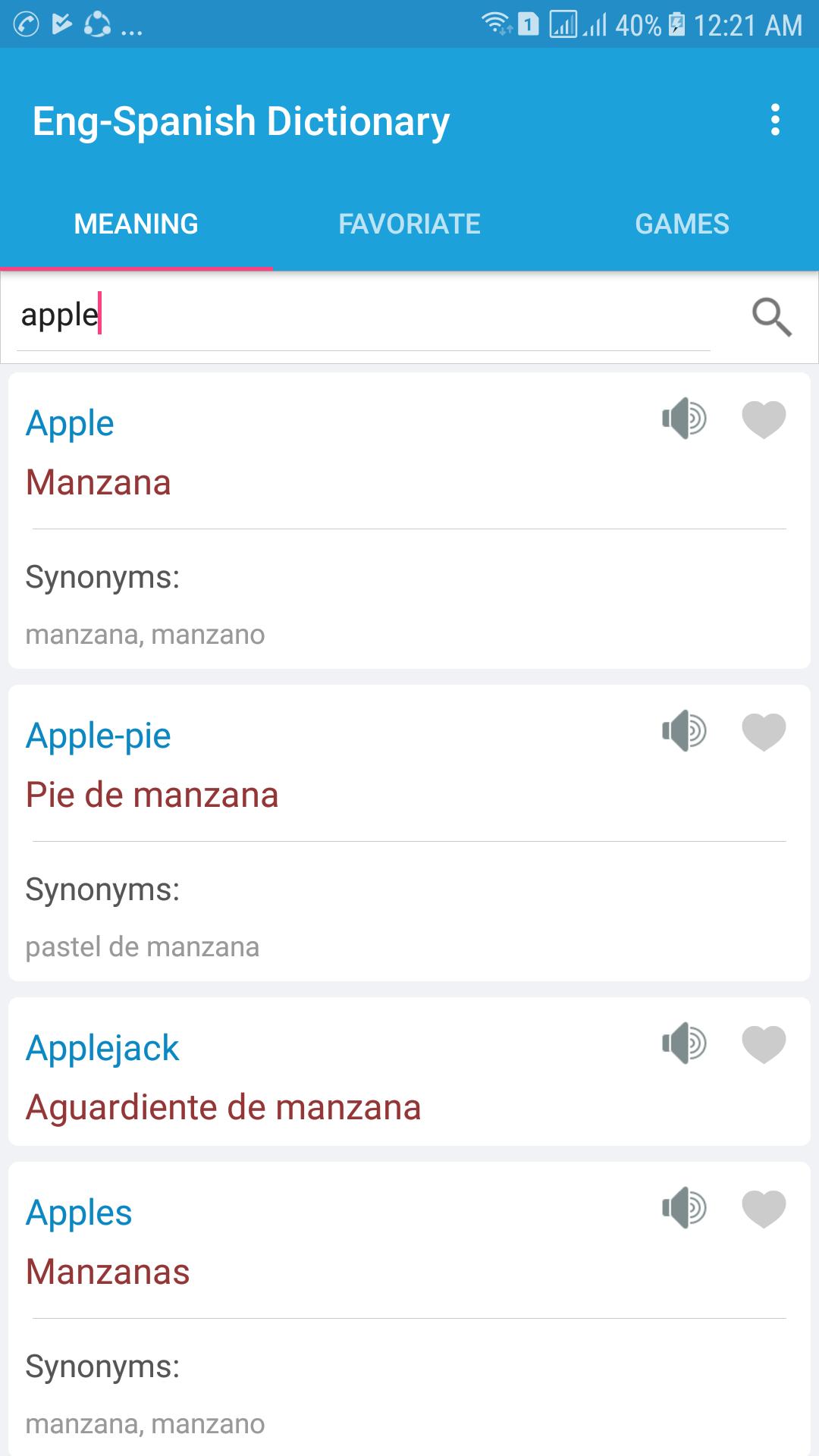This image captures a screenshot of a mobile webpage, titled "English-Spanish Dictionary" which is displayed in white text on a blue background at the top of the screen. Directly below the title, there is a navigation menu comprising several tabs: "Home," "Dictionary," "Favorites," and "Games," with the "Dictionary" tab currently selected.

In the main content area, the user has entered the word "apple" into the search field. The page presents the translation and related terms against a simple white background. The word "apple" is highlighted in blue for English and its Spanish translation "manzana" is highlighted in red. Additionally, several related terms and their translations are provided: "apple pie" translates to "pie de manzana," "apple jack" to "aguardiente de manzana," and "apples" to "manzanas." 

Below these translations, there are synonyms listed in black and gray text. Accompanying each term, small speaker icons are available to play the pronunciation of the words, offering an auditory aid for learners. This descriptive layout ensures that users can easily navigate and comprehend the dictionary entries, complete with visual and auditory features to enhance language learning.